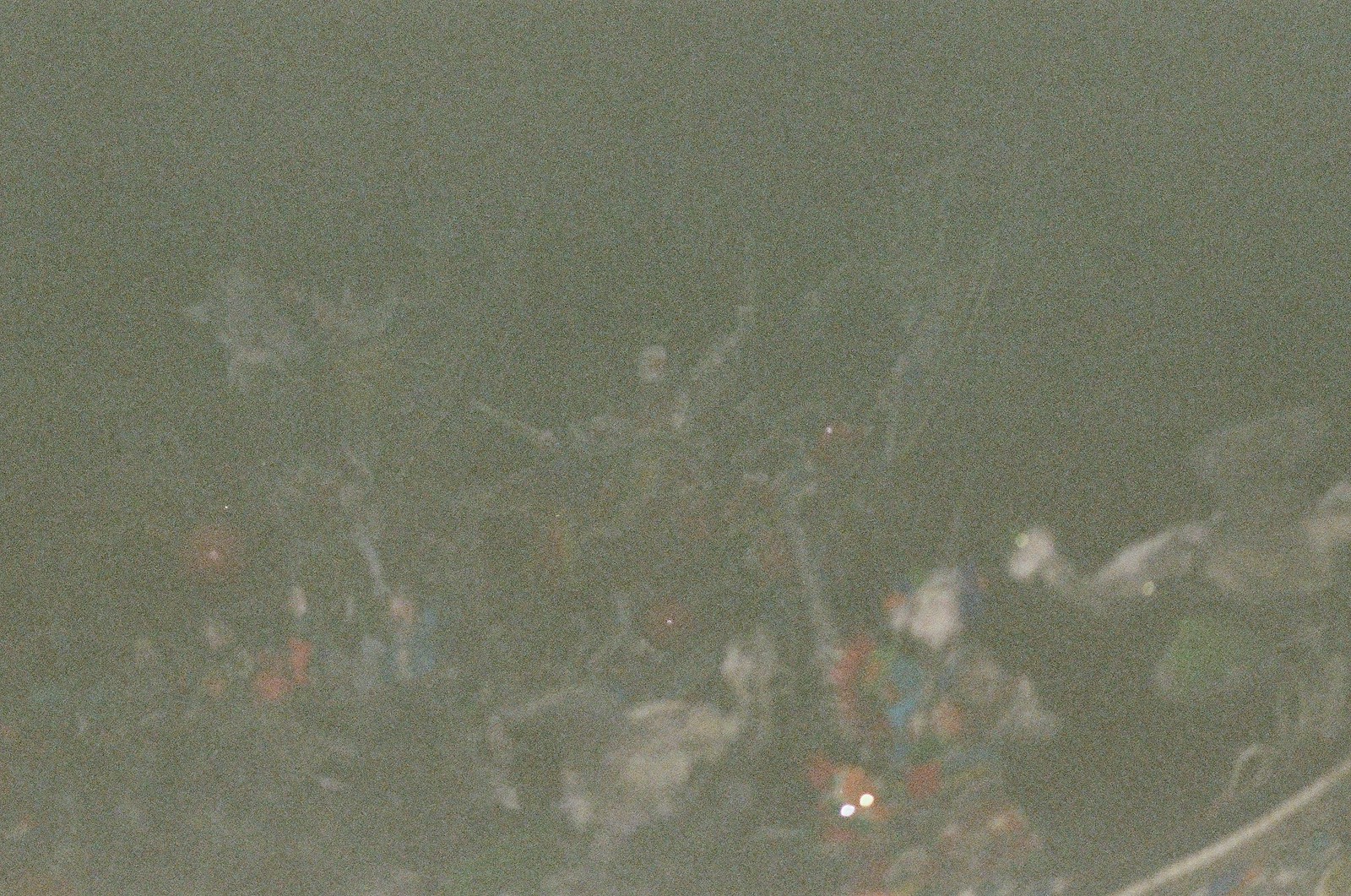The image is highly grainy and dark, presenting a challenging view of its contents. Predominantly, the top portion of the photo is enveloped in a black and grainy texture. On closer examination, faint orange glowing dots appear, primarily toward the bottom right, seemingly attached to a rounded orange figure that could be interpreted as fish eyes. The ground is speculated to be covered with rocks and various decorations or foliage, though specifics remain indistinct due to the quality of the image. Scattered across the scene are hues of gray, white, green, red, and blue, which might hint at the outdoor setting at night amidst wooded surroundings, or perhaps an artistic reflection or painting. Faint, blurry white or gray trim is noticed at the base in the corners. Despite attempts to discern the scene, the overall foggy, dark, and grainy nature of the image makes it difficult to pinpoint exact details, leaving much to the viewer's interpretation.